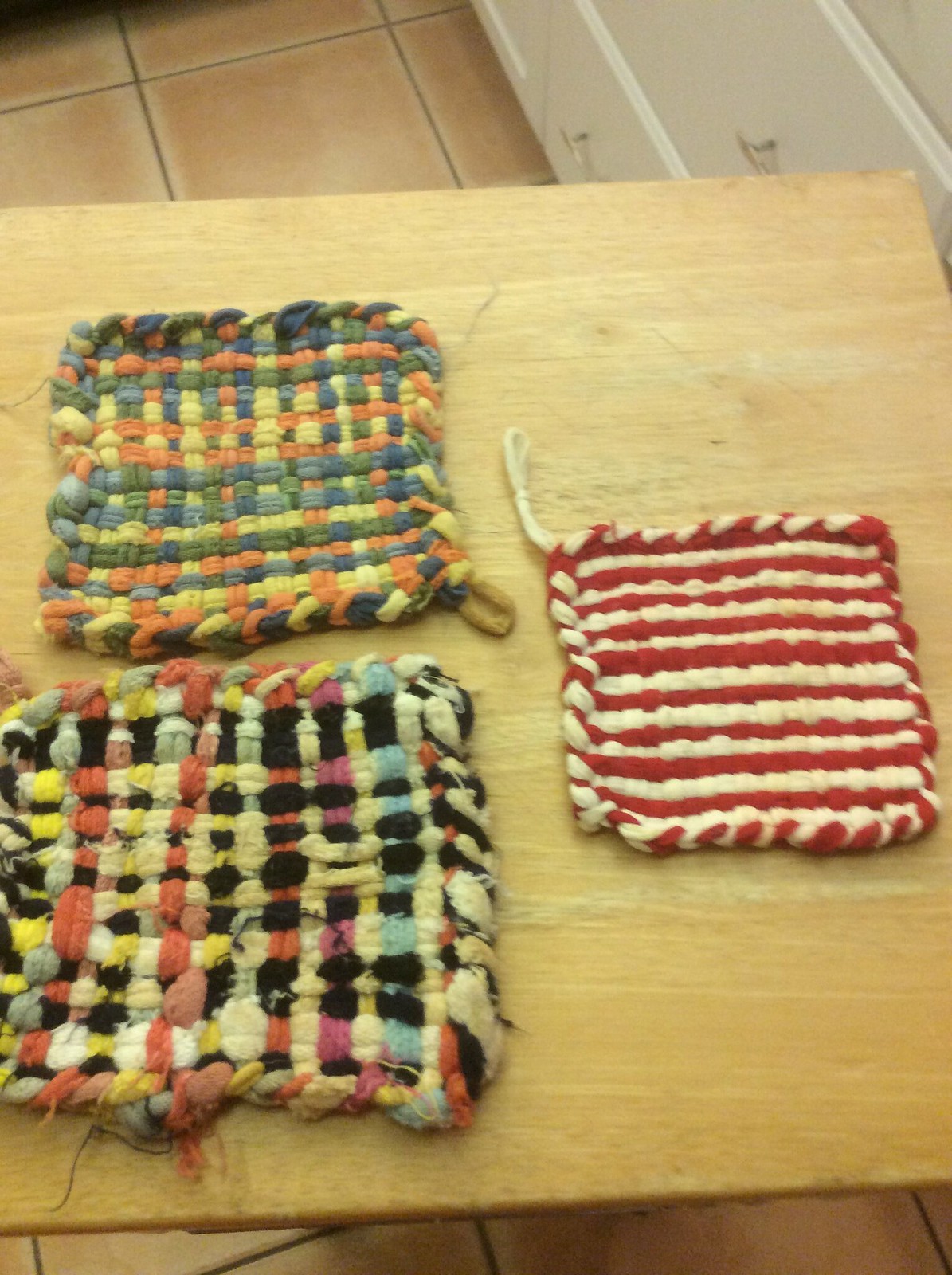The photograph displays the inside of someone's home, focusing on a light beige wooden table. On the table, there are three square-shaped, crochet-style hot pads, each with varying patterns and colors. The hot pad at the top showcases a mix of orange, yellow, blue, and green, creating a vibrant, multicolored design. To the right, there is a smaller hot pad featuring a classic red and white checkerboard pattern. The largest hot pad at the bottom flaunts an intricate combination of black with white, red, blue, yellow, and pink accents. The pads, designed for picking up hot kitchen items, lie against the warm, textured surface of the wooden table. In the background, you can notice a copper-colored tiled floor and white kitchen drawers, adding to the cozy domestic ambiance.